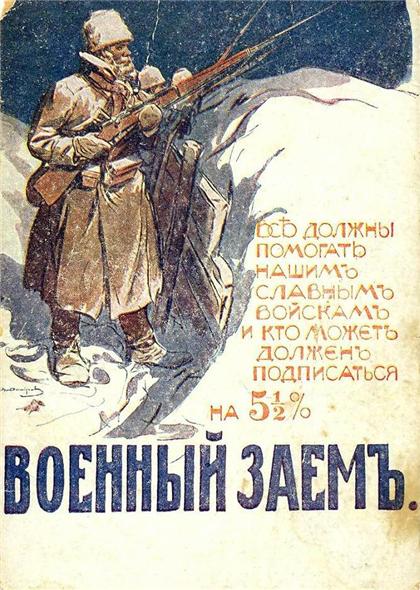This detailed war-themed poster features an evocative drawing set against a wintry backdrop. Dominating the top portion is an illustration of a man with dark brown skin, stationed behind a large snowbank on the right, amidst a snow-laden landscape. The man is clad in a heavy brownish-gray trench coat with the collar pulled up around his face, dark brown boots, and gray webbed mittens. He sports a gray helmet and is gripping a long brown firearm, positioned to the left and gazing rightward. A utility belt laden with various items girds his waist. Behind him, two other men are partially visible, wearing similar gray helmets. The sky overhead is painted a dark, ominous blue. Above the snowbank, orange text in an unreadable language, possibly Cyrillic, is clearly visible, along with a number stated as "5.5%". Below, larger all-caps text is printed in a dark blue font.